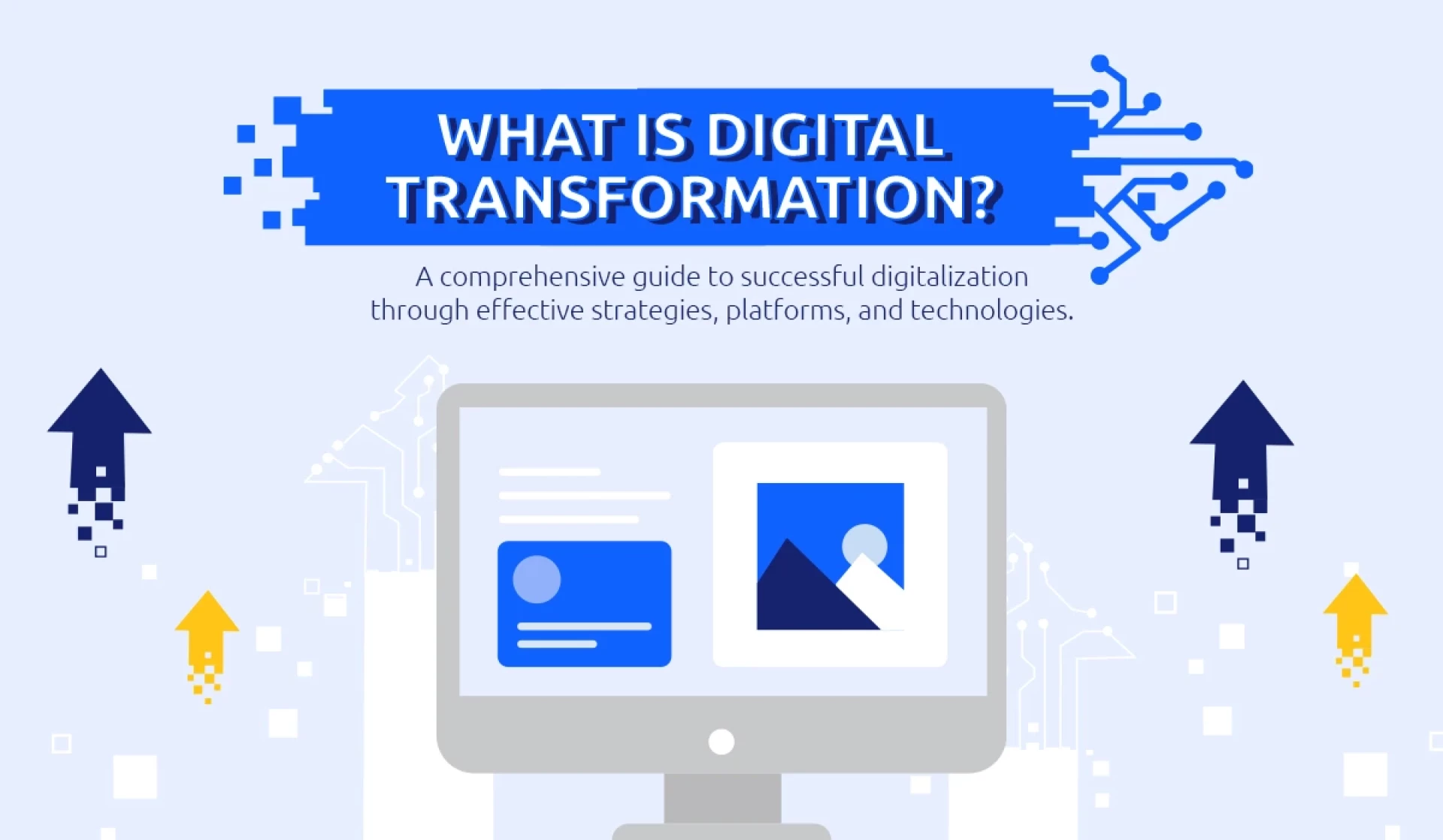The image features a light blue background with a prominent title at the top, "What is Digital Transformation?" written in white letters on a darker blue square with subtle networking graphics extending from it. Below this title, a subtitle reads, "A comprehensive guide to successful digitalization through effective strategies, platforms, and technologies." At the center of the image, there is a simple drawing of a computer screen displaying text and a picture of mountains. Surrounding the computer screen are various arrows pointing upwards: dark navy blue arrows on either side, smaller yellow arrows, and lighter white arrows, creating a sense of upward movement and growth. The overall design and color scheme give the impression of an early 2000s advertisement, possibly for a tech guide or an instructional infographic.